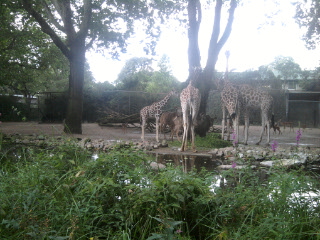In this small, color photograph, a group of at least four giraffes are featured in what appears to be a zoo exhibit. The image quality is somewhat degraded and blurry, but it's clear enough to depict a man-made environment. The ground, which may be concrete or cleared dirt, is bordered by what looks like a body of water—possibly a moat intended to keep observers at a distance from the animals. Various fences, possibly chain-link covered with green cloth, and some industrial structures can be seen in the background. 

Prominently, the giraffes are gathered around two main trees in the image, particularly a central tree with two large upward branches, and another tree to its left. Three of the giraffes have their heads down, seemingly engrossed in eating, while one appears smaller, likely a baby giraffe. There is also some green foliage in the foreground, adding a touch of natural greenery to the otherwise artificial environment. An unidentified animal partly obscured by one of the giraffes is also present, adding a hint of mystery to the scene.